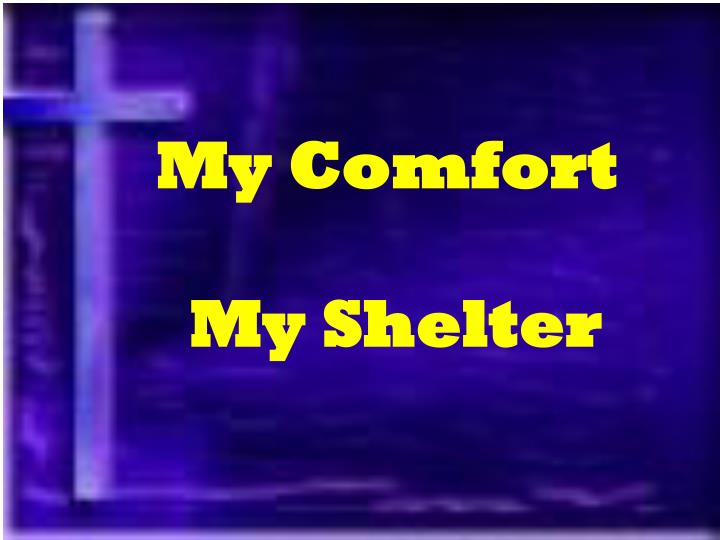This image resembles a still from a video, characterized by VHS-like artifacting, though this is only visible in the background. Predominantly, the background features various shades of purple and blue, with a hazy and blurry texture. The left side of the image showcases a tall, light purple Christian cross extending nearly from top to bottom. This large cross contrasts with the darker purple hues that dominate the rest of the background. 

In the center of the image, occupying the upper third and about 40% up from the bottom, are two lines of yellow block text. The text reads "My Comfort, My Shelter," with both the 'M' in "My" and 'C' in "Comfort" capitalized. This repeated format emphasizes central alignment and likely hints at a religious presentation, possibly a PowerPoint slide, as suggested by the structured and formal arrangement. The entirety of the image is framed by a white border, further enhancing its presentation-like quality.